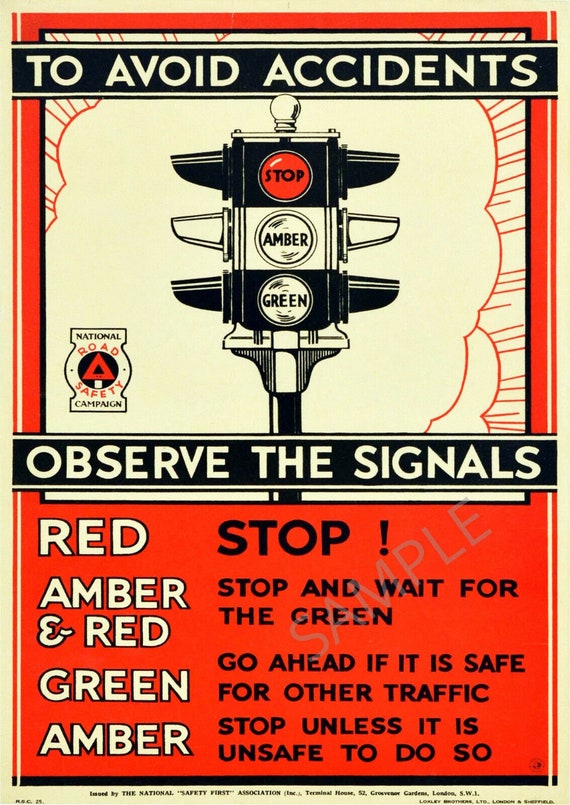This image depicts a vintage-style public service announcement poster aimed at promoting road safety. The poster features a beige border surrounding a predominantly reddish-orange background. At the top, a black bar bears the beige text "To Avoid Accidents." Below this, a large illustration of a traffic light shows its three stages: "Stop" in a red circle, "Amber" in a yellow circle, and "Green" in a green circle. The traffic light seems to have multiple visible sides, with the current light highlighted as red. Another black bar just below the illustration reads "Observe the Signals."

Towards the bottom of the poster, a detailed list provides traffic light rules. The left side of the list displays the words "Red," "Amber," and "Green" in white text with black outlines, while the right side contains the corresponding instructions in black text: "Red: Stop," "Amber: Stop unless it is unsafe to do so," and "Green: Go ahead if it is safe for other traffic." Additionally, a smaller illustration or icon is present in the bottom left corner, labeled "National Campaign for Road Safety." The background shading includes yellow borders accentuated by a red outline.